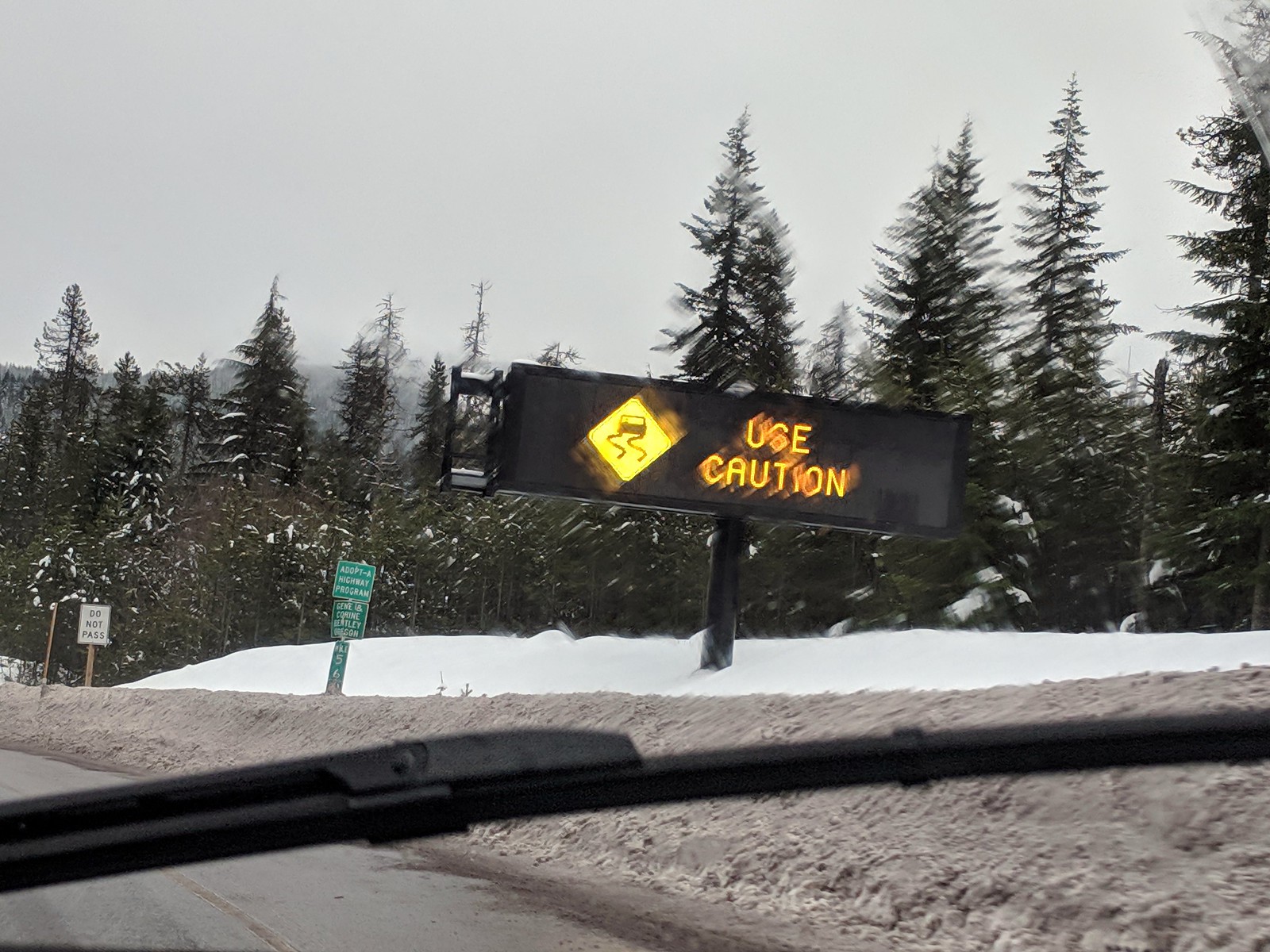The image appears to be taken from the interior of a car, looking out through the windshield. In the foreground, the windshield wiper is visible across the bottom half of the screen. The road ahead is flanked by dirty snow along the roadside, gradually transitioning to fresher, whiter snow as it ascends up the slopes. Fir trees, lightly dusted with snow, border the roadway. The sky overhead is a dull, overcast gray, suggesting ongoing snowfall.

Prominently displayed is a large black sign that reads "USE CAUTION," accompanied by a yellow warning icon depicting a car skidding, indicating slippery road conditions. Several other road signs are noticeable: green signs promoting the "Adopt a Highway Program," and another referencing regional information. There is also a signpost showing mileage or kilometer markers and a general warning sign stating "DO NOT PASS." In the distance, the landscape features gently rolling foothills dotted with fir trees, imparting a mountainous ambiance despite the absence of high peaks.